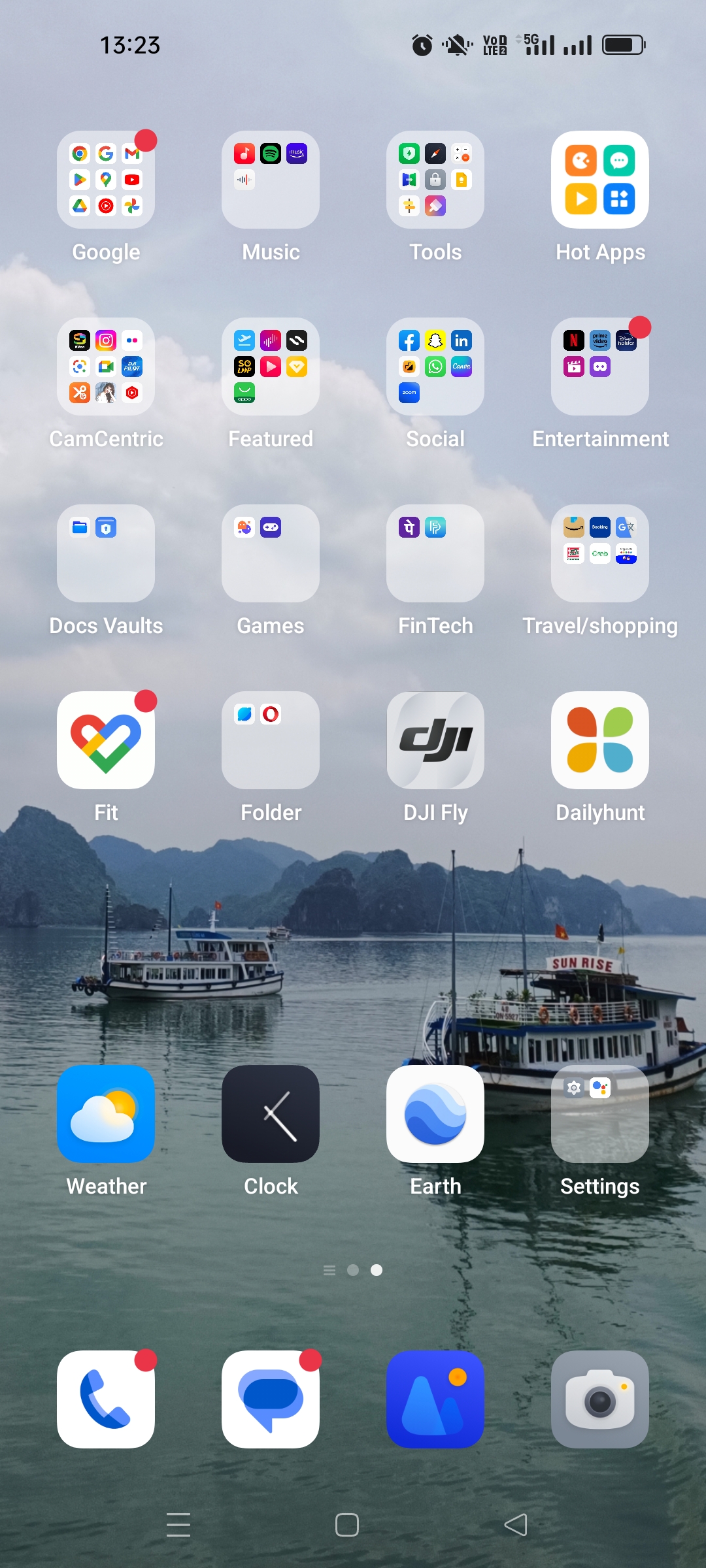This screenshot showcases a highly organized smartphone home screen, arranged meticulously into distinct app folders. At the top, the status bar displays various notifications and indicators, including a nearly full battery symbol and an alarm icon, which is depicted with a clock design. The time is shown in military format, reading 13:23 (1:23 PM).

The home screen features uniformly styled folders, each represented by a clear gray square containing a cluster of different colored squares. The top row folders are labeled "Google," "Music," "Tools," and "Hot Apps" from left to right. The second row includes "Cam-centric," "Featured," "Social," and "Entertainment." The third row houses "Dock Vaults," "Games," "Fintech," and "Travel Shopping." The bottom row contains folders named "Fit," "Folder," "DJ Fly," and "Daily Hunt."

The background image of the smartphone presents a serene lake scene, featuring two boats, adding a touch of tranquility to the meticulously organized home screen.